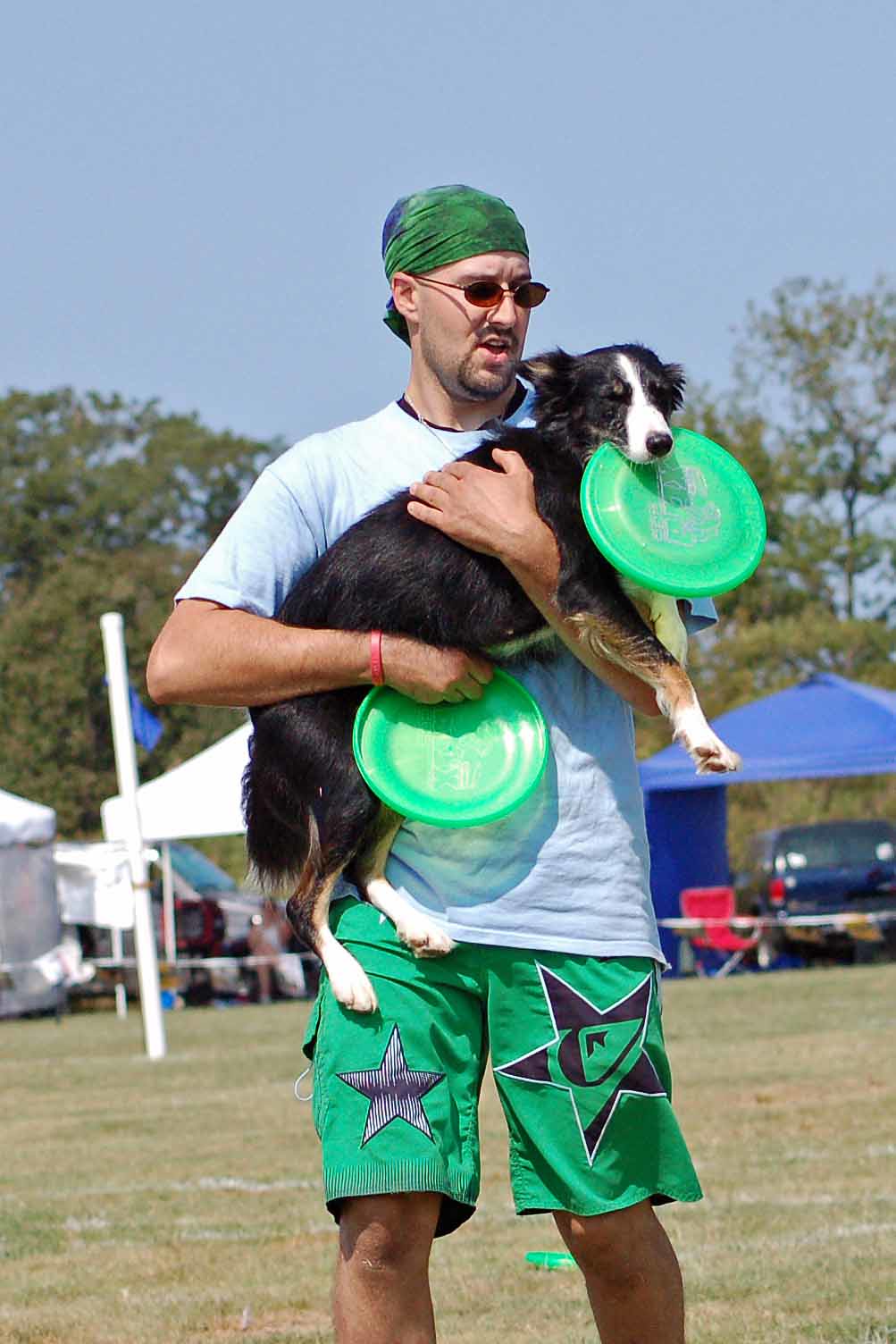This photograph captures a vivid outdoor scene set against a backdrop of a bluish-gray sky and green trees. In the middle of a grassy field, various tents are arranged, one being a blue canopy with a dark vehicle and a red chair inside it. Toward the left, a white tent stands near a conspicuous white pole. Additional tents and assorted objects appear in the blurred background.

In the foreground stands a tall Caucasian man in his 40s, with his hair pulled back by a green bandana. He wears a white short-sleeved t-shirt and green shorts adorned with black star designs. His right wrist sports a red rubber bracelet, and he is also wearing small round sunglasses. The man holds a black and white Border Collie with a distinctive white stripe around its muzzle and white feet. With his right hand, the man grasps a green Frisbee, while his left securely supports the dog under its chest. The dog, meanwhile, looks directly at the camera, holding another green Frisbee in its mouth. This dynamic and detailed image highlights both the serene environment and the playful bond between the man and his dog.